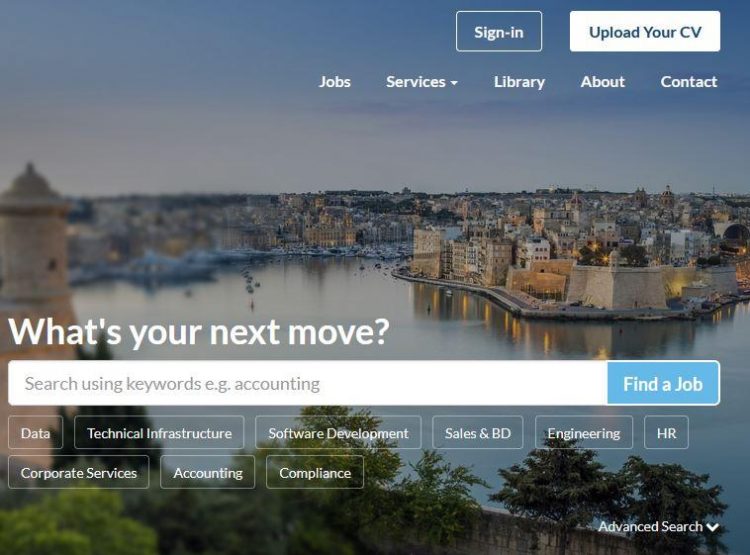This is a homepage for a website featuring a picturesque background that provides a welcoming ambiance. About a third of the way down, the backdrop showcases a clear, blue sky. On the left side, there is a prominent, brown tower extending from just above the skyline down to about an inch from the bottom of the image. Adjacent to this structure, slightly to the right, there is a stretch of thick trees occupying the bottom half, complemented by two additional trees to the right of the primary cluster, alongside a discernible concrete barrier. Below the expansive sky, the city skyline draws a horizontal line from left to center, about an inch down, and extends rightwards, descending roughly three inches into the water beneath. The water captures faint reflections of city lights, creating a serene effect.

In the upper right corner, a white tab with blue text prompts users to "Upload your CV". To its left, a blue rectangle bordered in white houses the "Sign In" button in white text. Directly below the CV tab, a white navigation bar reads, from right to left: "Contact", "Library", "Services", marked with an inverted white triangle, and "Jobs".

Positioned two-thirds down the page, bold white text poses the question "What's your next move?" directly above a long, white search bar. On the right end of the search bar, extending about two inches, a blue tab invites users to "Find a Job" in white text. Below the search bar are six tabs, followed by three additional tabs displaying varied information categories such as Data, Engineering, and HR. In the bottom right corner, a prompt for "Advanced Search" accompanied by a right-facing arrow provides further navigational aid.